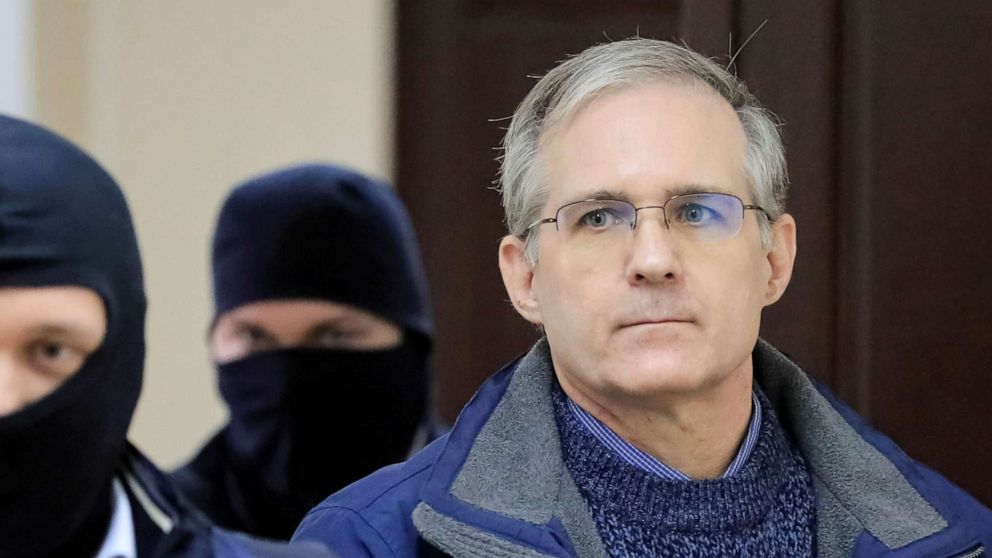In this photograph, the primary focus is an older Caucasian male, likely in his late 60s or early 70s. He has gray hair, parted to the left, with some patches of black. His eyes are gray and framed by semi-rimless glasses—rims on top, rimless on the bottom—and his expression appears serious, with lips pressed together. He's dressed in a layered outfit: a blue dressy shirt peeks out from under a thick blue sweater, which in turn is covered by a blue and gray jacket. To his right, two men appear, visible only from the shoulders up. They are wearing black ski masks that cover their entire faces except for their eyes, which reveal Caucasian skin underneath. The background features a mix of colors—white, beige, and dark brown—giving a hint of a wooden wall or paneling behind them.